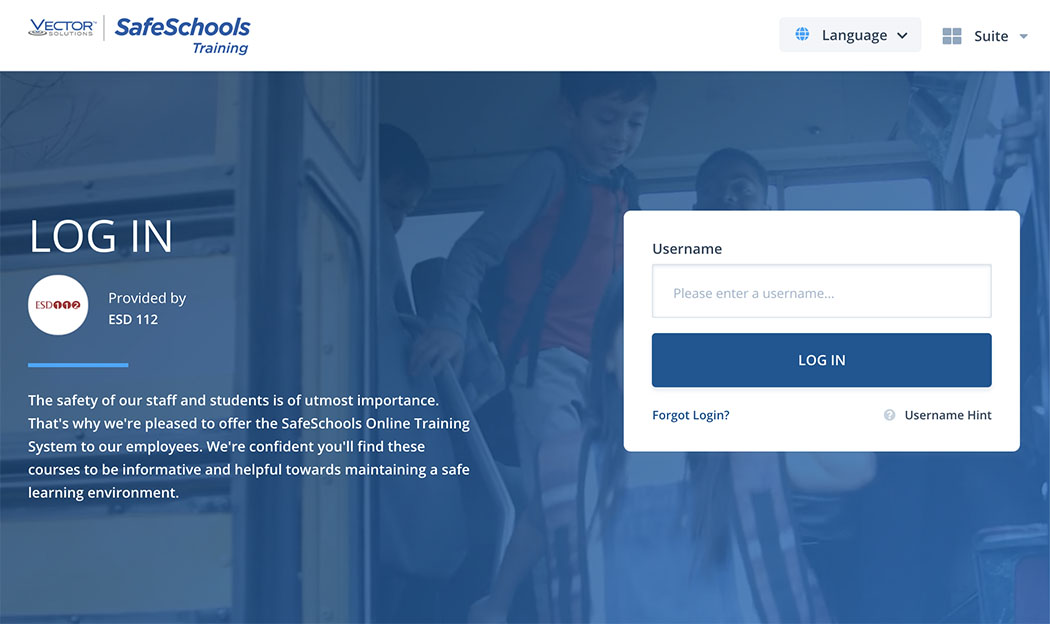This image is a carefully cropped screenshot of a web page from the Safe Schools Training system, a subsidiary of Vector Solutions. The company’s brand logo is prominently displayed in the top left corner, with a grey vertical line separating it from the blue text that reads "Safe Schools Training." On the top right of the page, there are dropdown menus to select the language and suite options for the user. The main focus of the web page is a login area, set against the backdrop of a photograph depicting children disembarking from a school bus. In the center of the page is a white rectangular box where users can enter their username, adjacent to a blue login button. Below this, there is explanatory text providing information about the system, emphasizing its role in ensuring the safety of staff and students through online training modules.